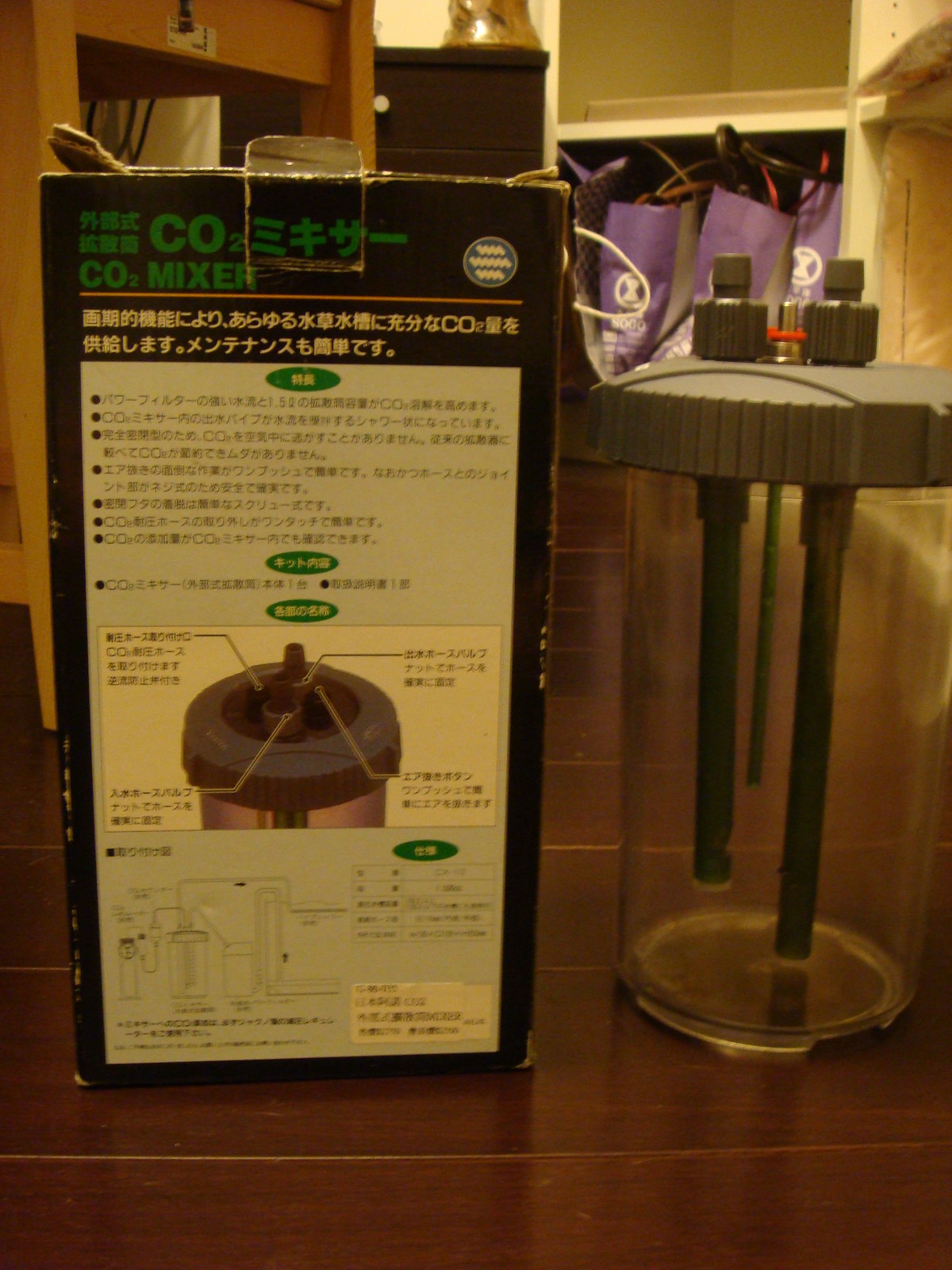The image depicts a CO2 mixer setup placed on a dark brown, horizontally-slatted hardwood floor in what seems to be a room, possibly a dressing room. The main component is a clear plastic or glass bottle with a dark gray cap, featuring three green straw-like objects and multiple hookups. To the left of the mixer is a vertically standing rectangular box, primarily light blue with a black top section, covered in Japanese text that seems to explain the product and its components, with 'CO2 mixer' being the only English text visible. Behind the box and mixer, there are shelves or cubbies holding purple bags intertwined with cords, along with a chair or stool and a dresser. The room is well-lit, adding clarity to the scene. The lack of reference objects makes it difficult to determine the exact size of the mixer.